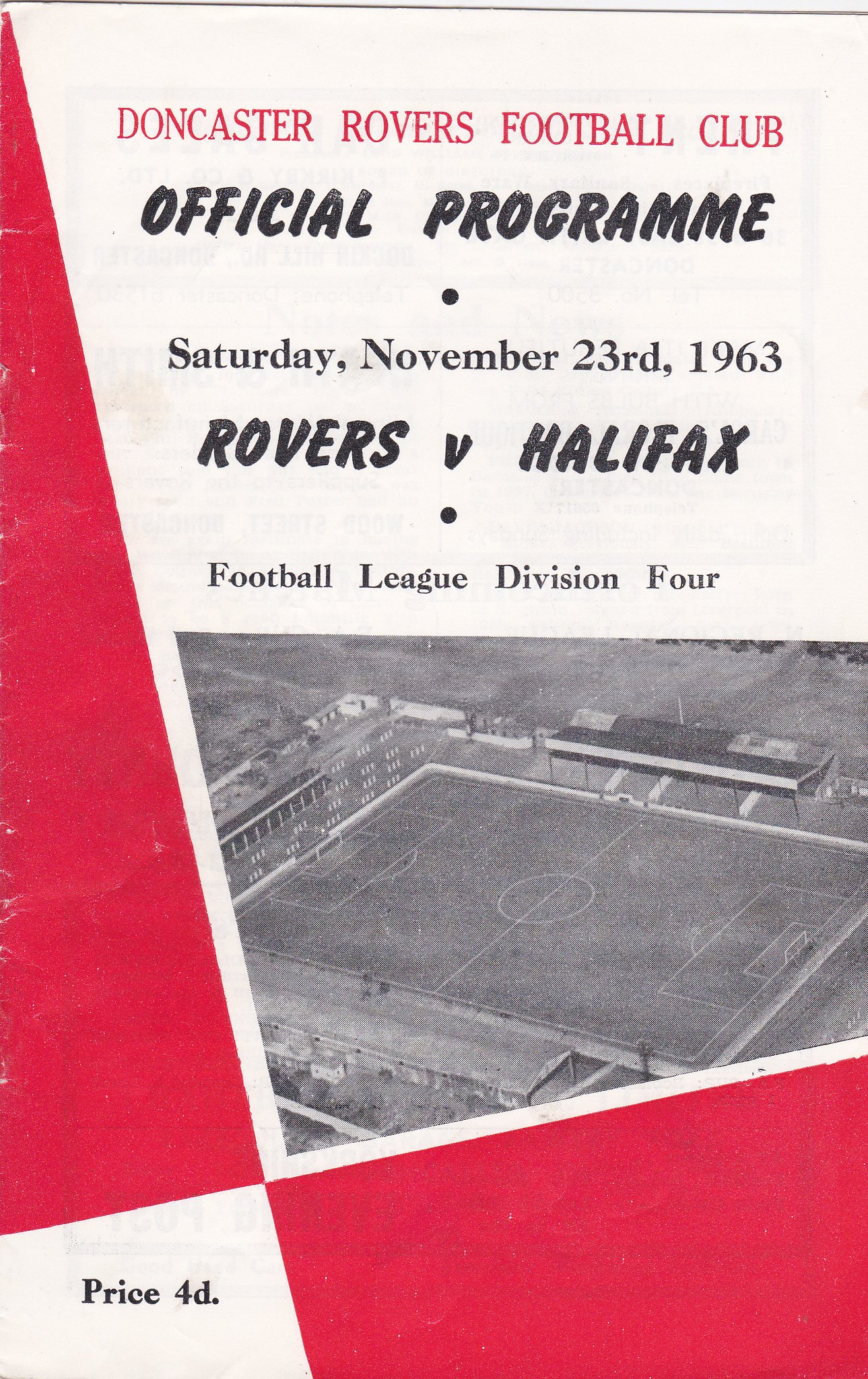The cover of the official game day program for Doncaster Rovers Football Club, dated Saturday, November 23, 1963, is printed in a striking combination of red and black ink. At the top, bold red text prominently displays "Doncaster Rovers Football Club," while directly beneath it, "Official Program" is printed in black. The date and match information, "Saturday, November 23, 1963 Rovers vs. Halifax, Football League Division 4," follows in black text. On the bottom left corner, the price "4-D" is indicated inside a small white box. The center of the cover features an angular aerial black-and-white photo of a soccer field or stadium. The design elements include an abstract red shape, resembling half a triangle extending from the top left to the bottom, intersecting with a red rectangular box at the bottom right.